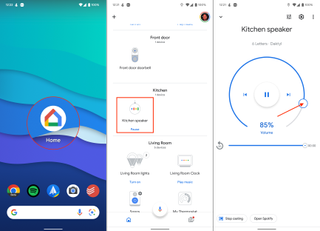The image showcases a composite of three screen captures from a digital device displayed side-by-side. 

The first screen capture on the left features the device's home screen. It is adorned with an aesthetically pleasing wave-design background comprised of gradients in green, blue, a darker shade of blue, and purple. Dominating the center of the screen is a white circle containing a triangular emblem, possibly an app icon. At the bottom of the screen lies the Google search bar, accompanied by a row of commonly used Google icons.

The second screen capture, centrally placed, primarily exhibits a white background, punctuated by various images and diagrams, suggesting either a webpage or a document. The central focus of this capture is a prominent red square, drawing immediate attention.

The third and final screen capture on the right maintains a white background. Within this frame, a blue circle is centrally positioned, featuring playback control icons including play, rewind, and fast forward. Above the circle, "kitchen speaker" is inscribed in black text, indicating the likely presence of media control options for a designated kitchen speaker.

Overall, the image provides a visual summary of different functionalities and interfaces available on the digital device, showcasing a home screen, a document or webpage, and media control for a kitchen speaker.